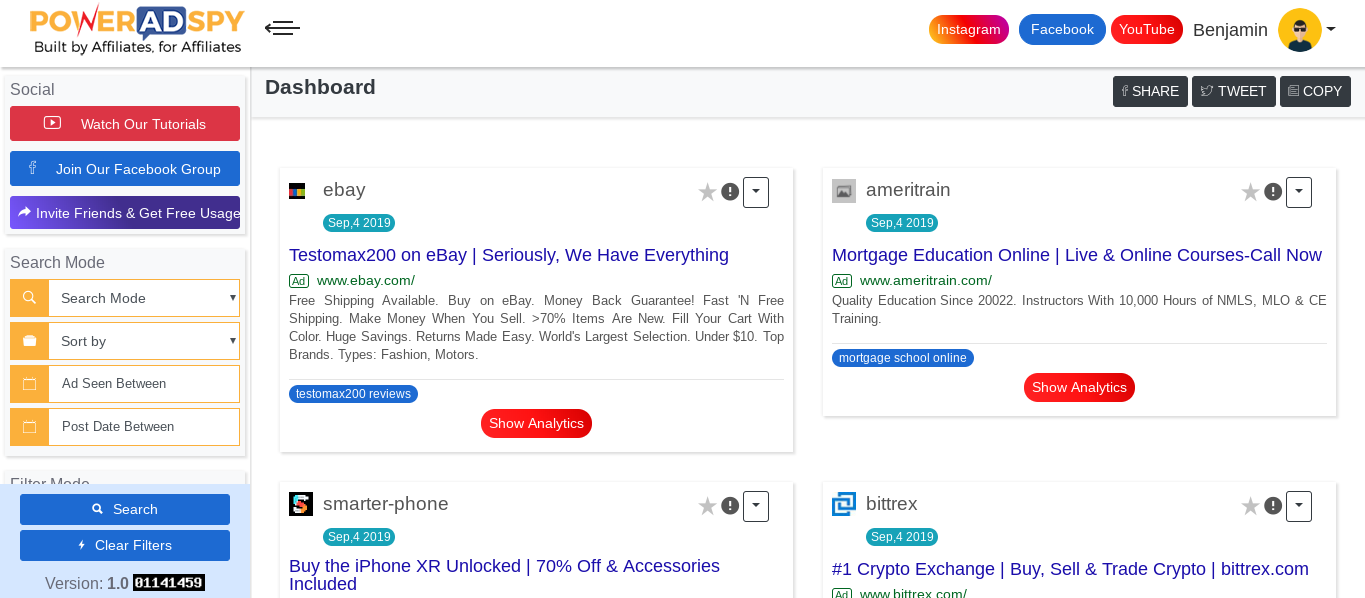This screenshot captures the interface of a website named "Power Ad Spy," designed specifically for affiliates by affiliates. The left-hand side of the page features a sidebar with multiple navigation options, starting with "Watch Our Tutorials," "Join Our Facebook Group," and "Invite Friends and Get Free Usage." This sidebar also contains a search button accompanied by options to "Clear Filters" and engage "Research Mode."

On the right-hand side, the top of the page displays three social media icons—Instagram, Facebook, and YouTube—next to a user profile section labeled "Benjamin," featuring a small, yellow avatar with a cartoon character. The main navigation header includes a "Dashboard" link along with options to "Share," "Tweet," and "Copy" the page.

The dashboard showcases four primary advertisement boxes. The first ad is for eBay, promoting "Testamax 200" with the tagline “Seriously, we have everything” in purple text. This ad is accompanied by a blue banner and a red oval button labeled "Show Analytics." The second ad is for "Ameritrain," highlighting "Mortgage Education Online" with live and online courses underlined by a blue banner stating "Mortgage School Online" and another red "Show Analytics" button.

Only partially visible at the bottom are two additional ads: one for "Smarterphone," focusing on an iPhone, and another for "Bitrex," centering on cryptocurrency. Despite being cut off, these ads contribute to the website’s comprehensive display of various affiliate campaigns.